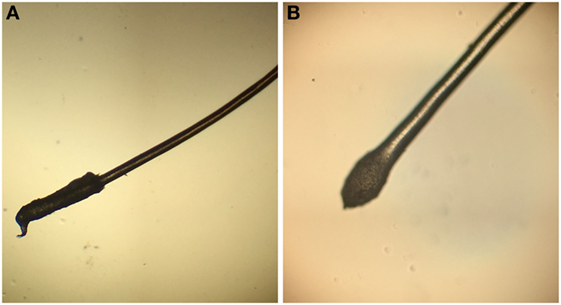The image consists of two closely-up, high-resolution microscopic photographs labeled A and B, intended for forensic evidence analysis. Both images display hair roots against distinctly light backgrounds, evoking a professional forensic examination setting.

Image A, situated on the left, depicts an anagen hair root characterized by a long, tapered sheath. The background is a very dark cream color, accentuating the hair's details. The hair root in this image extends diagonally from the top right to the bottom left corner, displaying a lush, black, fluffy end.

On the right, image B shows another type of hair root, this time with a bulb root. It features a brown stem tinged with a lighter cream stripe, culminating in a smaller, brownish, fluffy end. The photograph's amber background further highlights the contrast and subtleties of the hair's structure.

The photographs are neatly positioned side by side in a portrait orientation, divided by a white line, and illuminated by a bright light source that enhances the texture and reflective qualities of the hair strands. The images, differing in background color and hair root morphology, resemble close-up views under a microscope and are indicative of typical evidence used in crime scene investigations.